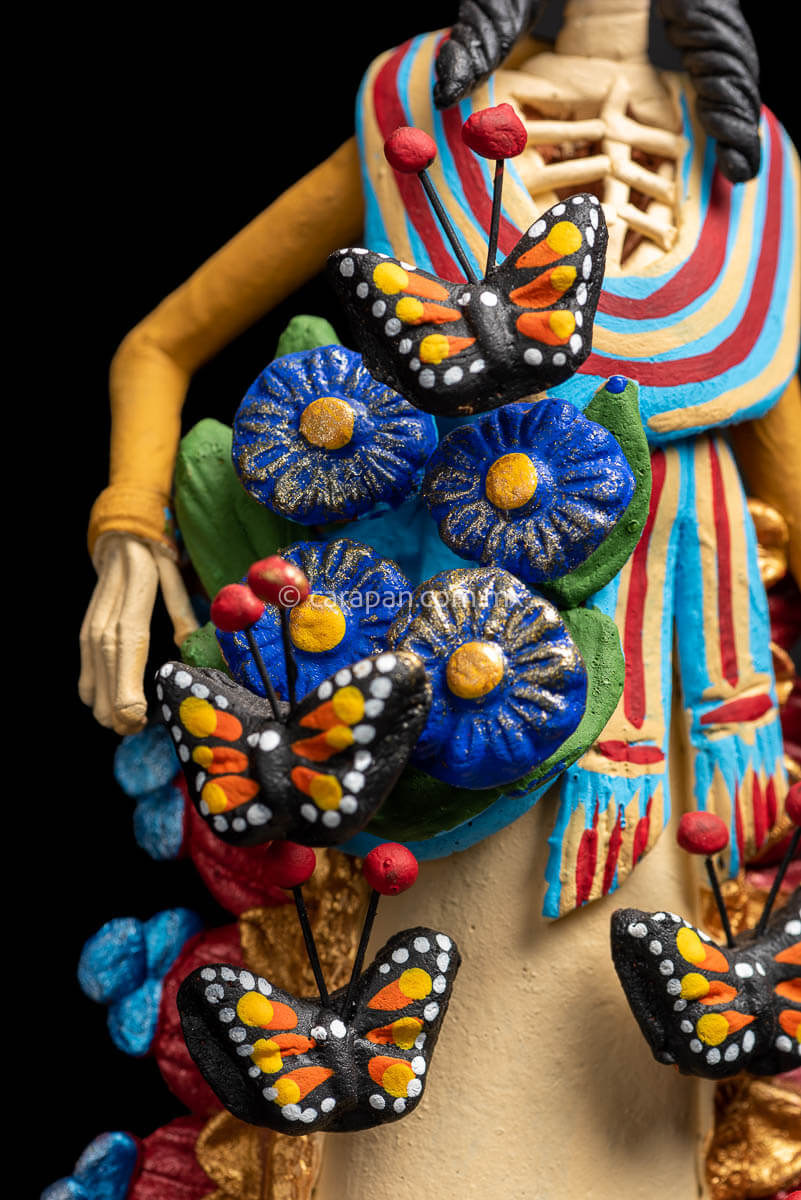This close-up photo captures a detailed view of a statue of a woman, sculpted from ceramic material. The image frames the figure from her neck down to just below her knees, showcasing her attire in vivid detail. The woman is adorned in an ivory-colored dress, accompanied by a vibrantly colored scarf in shades of red, blue, and ivory draped around her neck and hanging down the front. Her black hair gracefully curls over her shoulders, though her face is not visible in the image.

On her right side (viewer's left), she is flanked by four large blue flowers with yellow centers. Below these flowers, there are two black-colored butterflies, and an additional black butterfly on the left side. The butterflies are detailed with intricate orange and yellow patterns and feature notable red ball-tipped antennae. Her skeletal form is evident, with both her hands and chest displaying exposed bones rather than skin. Additionally, her right hand seems to be holding an elaborate flower, further enhancing the statue's ornate appearance.